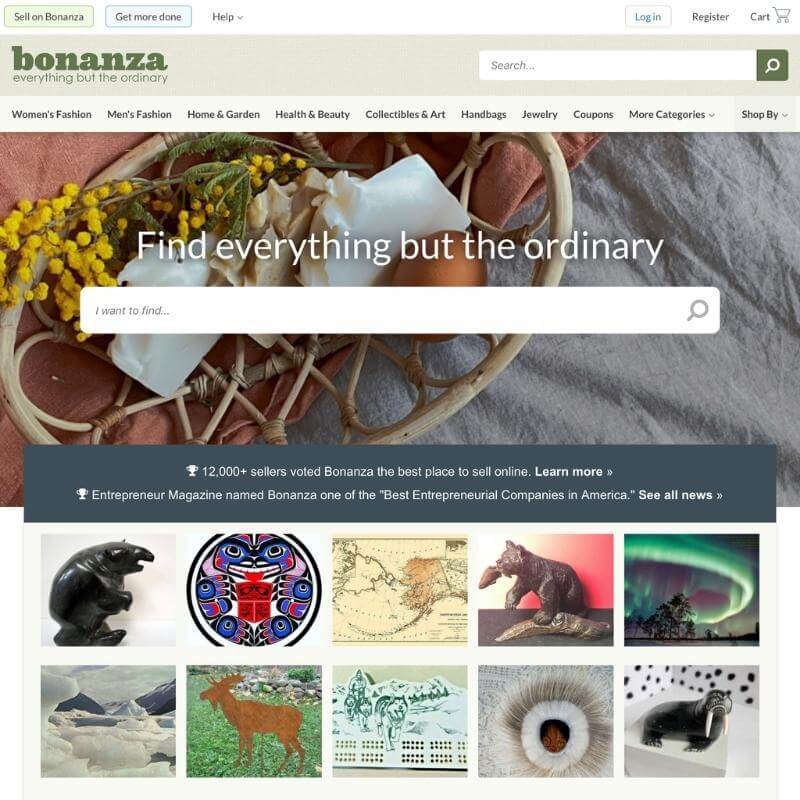This screenshot captures the homepage of the online marketplace website, Bonanza. At the very top of the page, there is a green navigation bar featuring options such as "Sell on Bonanza," "Get More Done," and "Help." On the right side of this bar, users can find options to log in, register, and view their cart, which is indicated by a shopping cart icon.

Centered below this navigation bar is the Bonanza logo, adorned with the tagline "Everything But The Ordinary," and accompanied by a prominent search bar. This search bar allows users to easily find specific items they're looking for.

Directly beneath the logo and search bar is a horizontal menu showcasing various categories including "Women's Fashion," "Men's Fashion," "Home and Garden," "Health and Beauty," "Collectibles and Art," "Handbags," "Jewelry," "Coupons," and a "More Categories" drop-down arrow. Additionally, there is a "Shop by Category" drop-down arrow offering further navigational ease.

The main visual content of the homepage features a large, inviting background image displaying baskets filled with various items such as flowers, leaves, and textured fabrics. Overlaid on this image is a prominent search box with the placeholder text "I want to find" and a search icon. Above the search box, the tagline "Find Everything But The Ordinary" is prominently displayed, reinforcing Bonanza's unique branding.

Below this central image, there is a dark gray bar highlighting accolades and announcements. Notably, it mentions that "12,000+ sellers voted Bonanza the best place to sell online" and that Entrepreneur Magazine named Bonanza one of the "Best Entrepreneurial Companies in America." Users are invited to "See all news" for more details.

The page also includes a trophy icon and a section for featured items. Overall, the layout is clean and visually appealing, with a slight amount of clutter. However, the use of large, vibrant background images creates an inviting atmosphere. The navigation and search options are clearly presented, making it easy for users to explore the site.